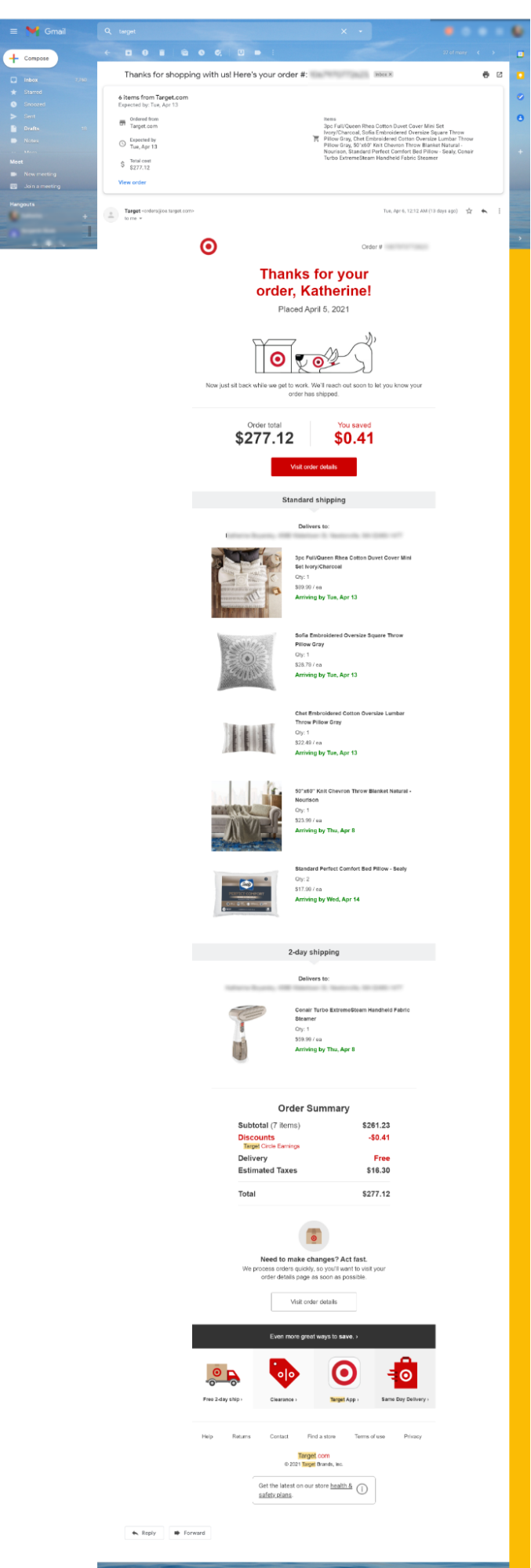The image displays a screenshot of an order confirmation webpage on a computer, presumably from the Target website, as indicated by the prominent red Target logo. Although the text on the page is not fully legible due to its small size, several details can be discerned. On the left side of the page, there are dropdown menus categorized under various headings.

At the top of the main section, in black text, it confirms the order with a message that reads, "Thanks for your order, Catherine," suggesting a personalized order confirmation. Below this message, there is an illustration of a box with the Target logo accompanied by a dog bowing towards the box, emphasizing the brand's recognizable mascot.

To the left of the box illustration, the figure "277.12" is displayed, likely revealing the total cost of the order. Below this, it mentions a savings of 41 cents. Underneath the figure, there is a prominent red bar followed by a gray bar with unreadable text.

Further down, there are images showcasing the purchased items. The first image appears to depict a pillow, with the second and third images also clearly representing pillows. The fourth image might be a throw, though it is somewhat ambiguous, and the final image is indiscernible at this size.

Another gray bar follows these product images, leading to another merchandise image that is too small to identify clearly. At the bottom section of the page, "Order Summary" is displayed in red, detailing the savings and order specifics in black text.

Finally, the bottom of the webpage contains a black bar with icons of a truck, price tag, the Target logo, and a red box, likely providing quick access to additional features or services related to the order.